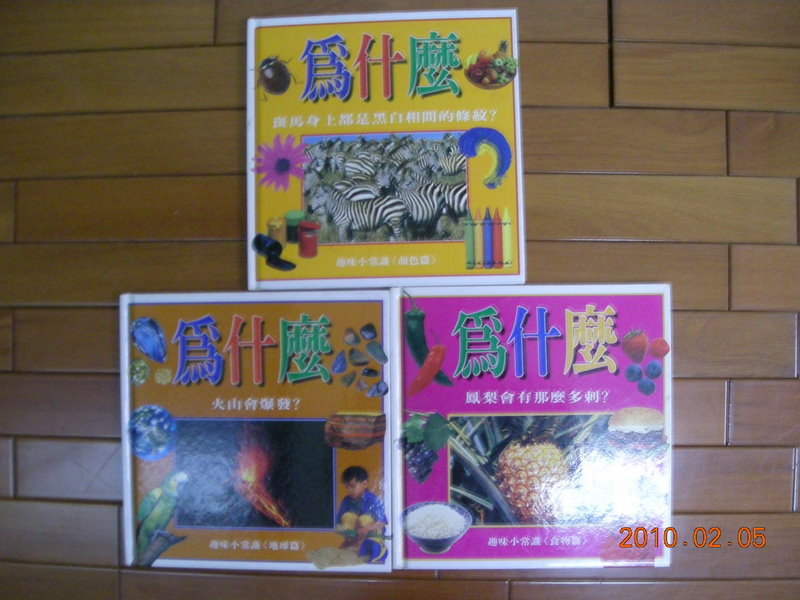In the image, there is a light brown wood grain surface, which could either be a wall if viewed from a standing position or a table if the camera is positioned above. On this surface, three distinct covers lie flat, likely children's books due to their vibrant and illustrative designs. The texts on these covers are written in what appears to be Chinese or Japanese characters.

The covers are each of a different color but share a similar artistic style. The topmost book has a yellow cover featuring an image of zebras, a pink flower to the left, jars of paints, and multiple colored crayons (green, yellow, blue, red, and mustard) in the bottom right corner. The text is multicolored, enhancing its playful appearance.

The book positioned at the bottom left has a brown cover and depicts a little boy in the lower left corner, a small bird in the lower right corner, and an illustration of the planet Earth in the upper right corner.

The book on the far right has a hot pink cover. It shows a pineapple in the center, a bowl of rice in the lower left corner, and a bunch of grapes in the upper left corner. In the bottom right of the image, a date is visible, marking "2020-02-05," which indicates February 5th, 2020, possibly related to when these books were published or released.